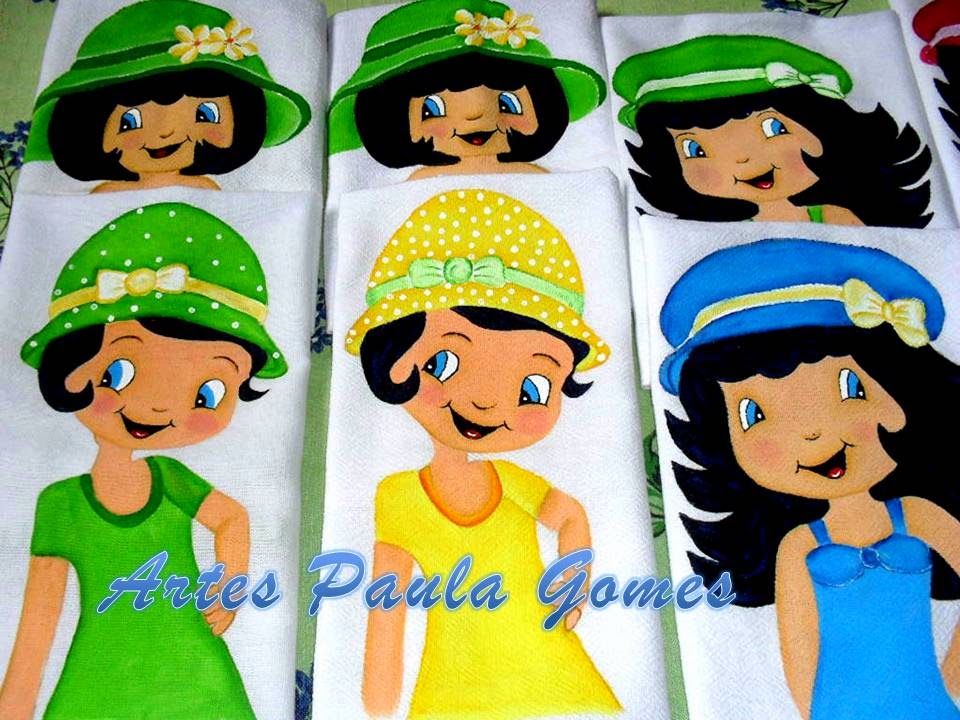The image features a grid of six cartoon girls arranged in three rows and two columns. Each cartoon girl is depicted on a different beach towel, making for a total of six towels. At the top, there are three girls with distinctive green hats adorned with yellow flowers, white ribbons, or bows, and they all share blue eyes and short black hair styled in either bobs or pixie cuts. The first girl in the bottom row is dressed in a green dress with a matching polka-dot hat featuring a white bow. The second girl, wearing a yellow hat with white polka dots and a coordinating yellow dress, has super short black hair and blue eyes. The final girl of the bottom row has long fluffy black hair, blue eyes, and is attired in a blue dress with a blue hat that includes a yellow ribbon. The visible text at the bottom of the image, printed in blue letters with a white outline, reads "Arte Paula Gomes."